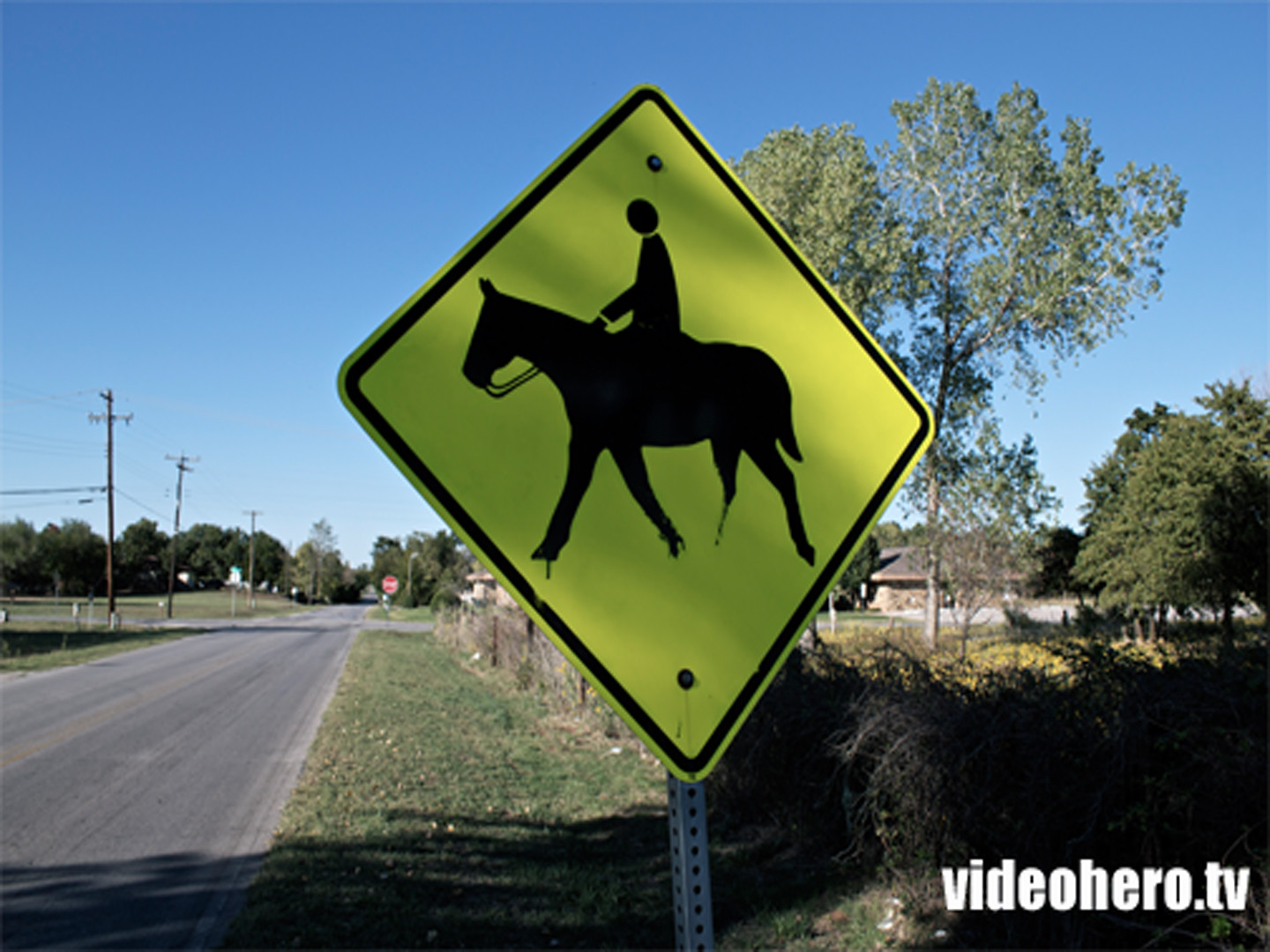The image captures a serene country road scene framed by nature and cautionary signage. A yellow diamond-shaped sign, mounted on a perforated metal pole, features an illustration of a horse and rider, indicating the presence of equestrian activity in the area. To the right of the sign, a rustic fence, overgrown with vines, stretches into the distance, adding to the rural ambiance. On the bottom right corner, the text "videohero.tv" is visible, likely indicating the source or artist of the photo.

The road itself, a quaint two-lane path, extends diagonally to the left, leading the viewer's eye towards the horizon. In the distance, several electrical poles line the pathway, while a prominent red stop sign punctuates the roadside. Surrounding the road, lush trees tower over a brick building with a brown roof, partially obscured by foliage. White fences dot the landscape, contributing to the overall pastoral charm of the scene.